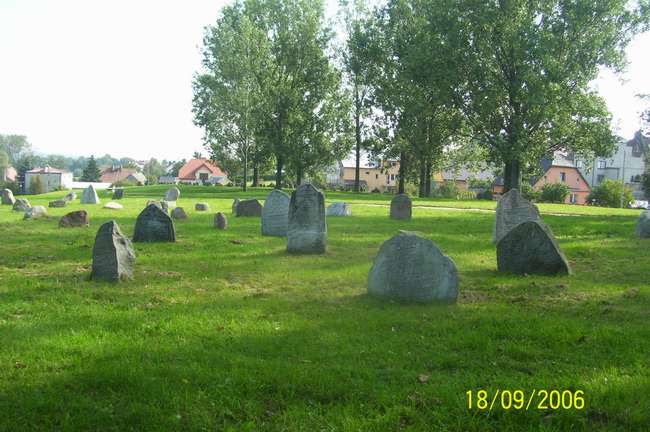This photograph shows an old cemetery captured on a bright day, as indicated by the white sky. The bottom right corner bears a date in yellow text: 18-09-2006. The graveyard features a flat, lush expanse of green grass scattered with about 25 headstones, many of which are large, irregularly shaped boulders in varying shades of gray, brown, and red. While some of these stones have inscriptions carved into them, others appear as simple, round boulders without visible text. In the background, there are houses with red roofs and tan sides, as well as tall trees with green leaves, contributing to the serene atmosphere of the scene.